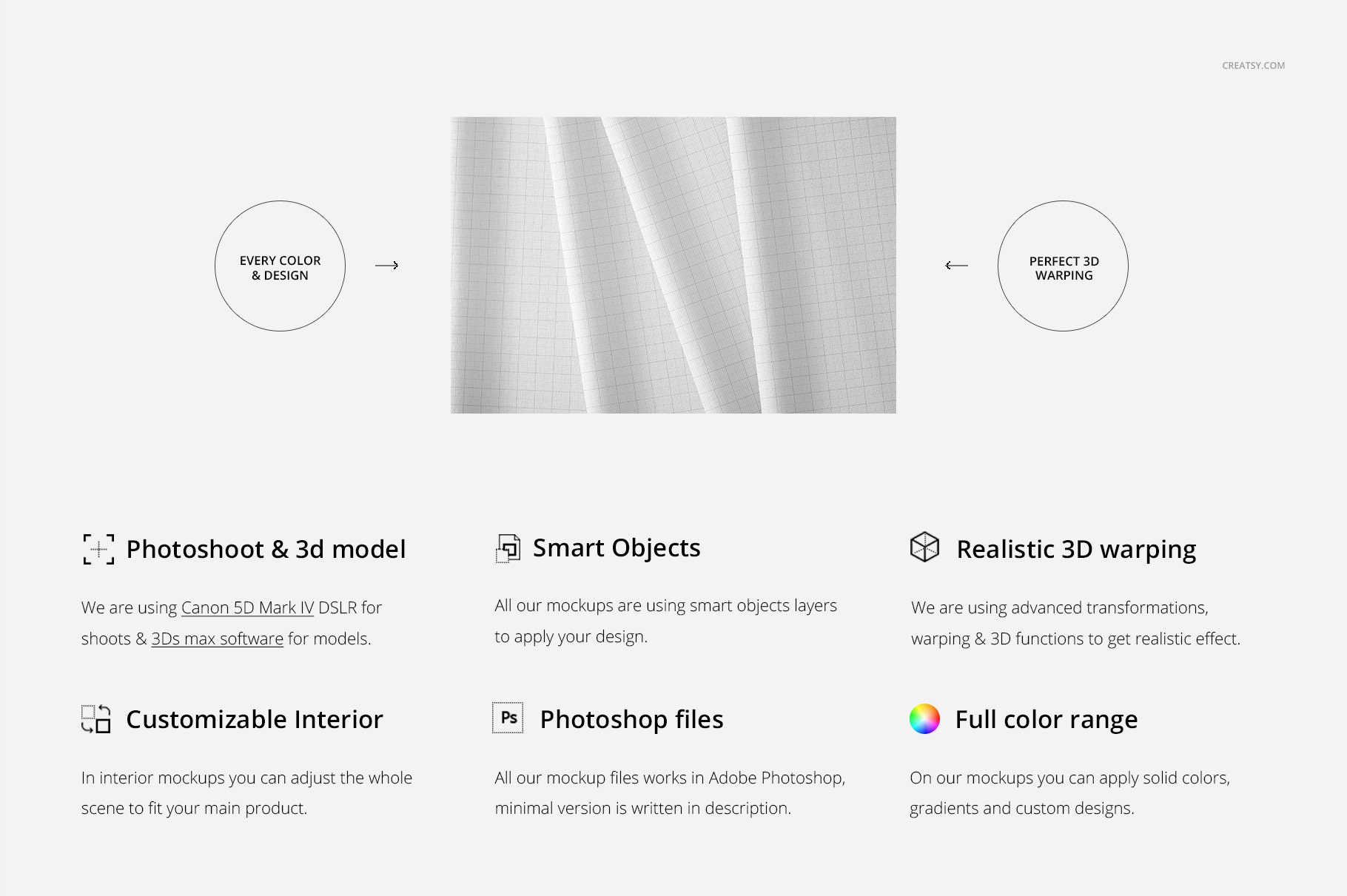This landscape-oriented image showcases a text box from what appears to be a website's product page, set against a gray background. The rectangular text box is slightly longer than it is tall. At the top, there's a faint watermark featuring the website "create seed.com."

At the center near the top of the text box, there's a photograph of a gray linen fabric with white accents, characterized by a grid or checkered pattern formed by intersecting vertical and horizontal lines, creating tiny squares. The linen, possibly curtains, shows some natural folds. To the left of this image, a black circle with white text contains the words "every color and design," pointing to the linen. Another circle with the text "perfect 3d warping" has an arrow pointing left.

Below this section, there are three columns, each containing two feature headers and descriptions, accompanied by representative icons. The headers from left to right read: "Photo Shoot & 3D Model," "Smart Objects," "Realistic 3D Warping," "Customizable Interior," "Photoshop Files," and "Full Color Range." Descriptions beneath each header provide further details on the features offered.